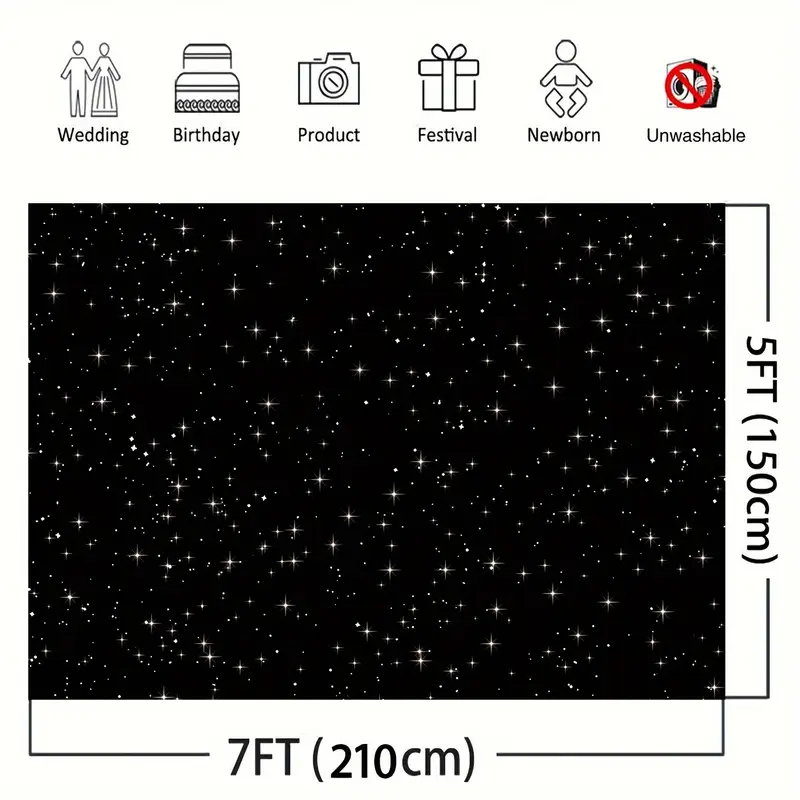This image appears to be an advertisement, potentially for a website, featuring a starry night sky theme. At the top, there are six icons, each representing different categories: a couple for weddings, a two-tiered cake for birthdays, a camera for products, a gift box for festivals, a baby for newborns, and a washing machine with a red "X" for unwashable items. Below these icons, the words "wedding," "birthday," "product," "festival," "newborn," and "unwashable" are displayed from left to right. 

The main section of the image showcases a black rectangular space scene scattered with tiny, sparkling white stars, providing a visually striking backdrop. Below this star-filled rectangle, the text "7FT 210CM" is prominently displayed, while the right side of the image features sideways text reading "5FT 150CM." The overall design of the image, with its blend of detailed icons and celestial motif, lends itself to an engaging and visually appealing advertisement or promotional material.